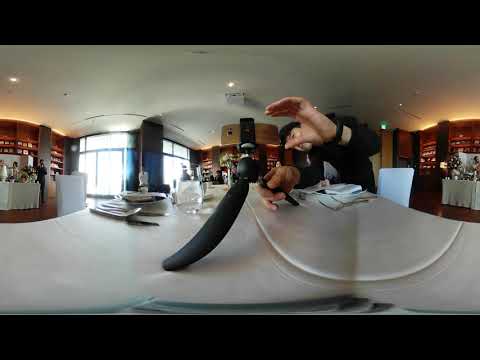In this distorted fisheye image, we observe a young man dressed in a black long-sleeved outfit, seated at an elegantly set white table in what appears to be a refined restaurant or event venue. The table is adorned with plates, silverware, and clear glasses filled with water, exuding a Michelin star ambiance. The man is positioned centrally, with his hands in a c-shaped grip around a sleek, black, blade-like object that extends towards the camera. His other hand reaches towards the object, suggesting he might be handling intricate equipment, possibly a tripod.

The background reveals deep brown, oak-like walls lined with shelves that host various products. To the far left and right, there are additional tables draped with white tablecloths, hinting at a possible buffet setup. The left side of the room features expansive windows that allow natural light to flood in, while the ceiling, primarily white, is warmly illuminated by amber-yellow lighting from the sides. The entire scene is slightly warped, giving it a surreal, curved appearance, enhancing the mystique and elegance of the setting.